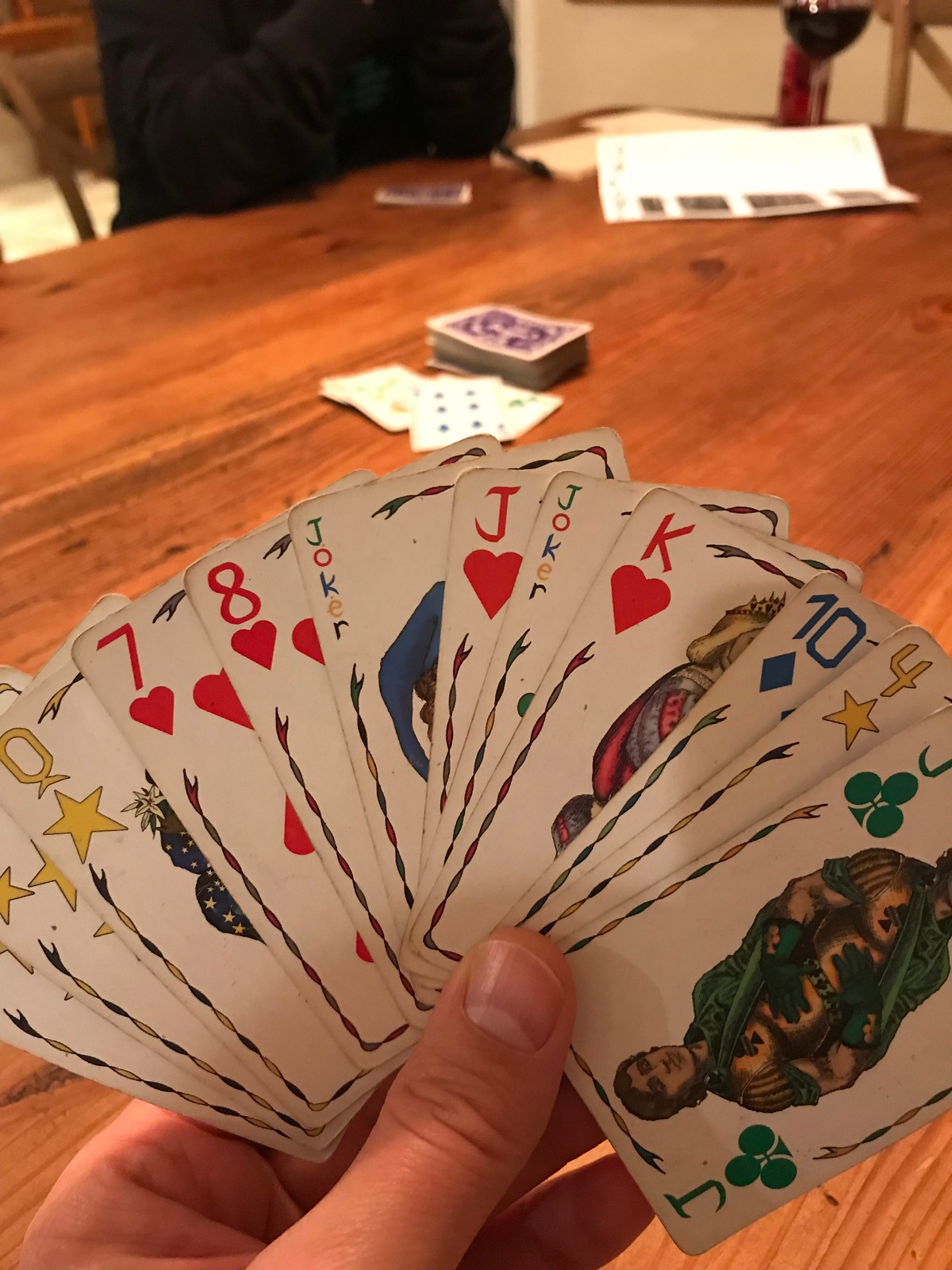The color photograph captures a close-up of a human hand holding a spread of 12 playing cards, including a Jack, a Four, a Ten, a King of Hearts, a Joker card, a Jack of Hearts, another Joker card, an Eight of Hearts, a Seven of Hearts, a Queen with a star symbol, and two additional cards, one also marked with a star. The background reveals a well-worn deck of cards and some discarded ones on a table, suggesting an ongoing game. A white piece of paper, likely for keeping score, lies nearby. Another player, wearing a dark shirt, is partially visible, sitting at the table with cards facing down, showing the competitive nature of the scene.